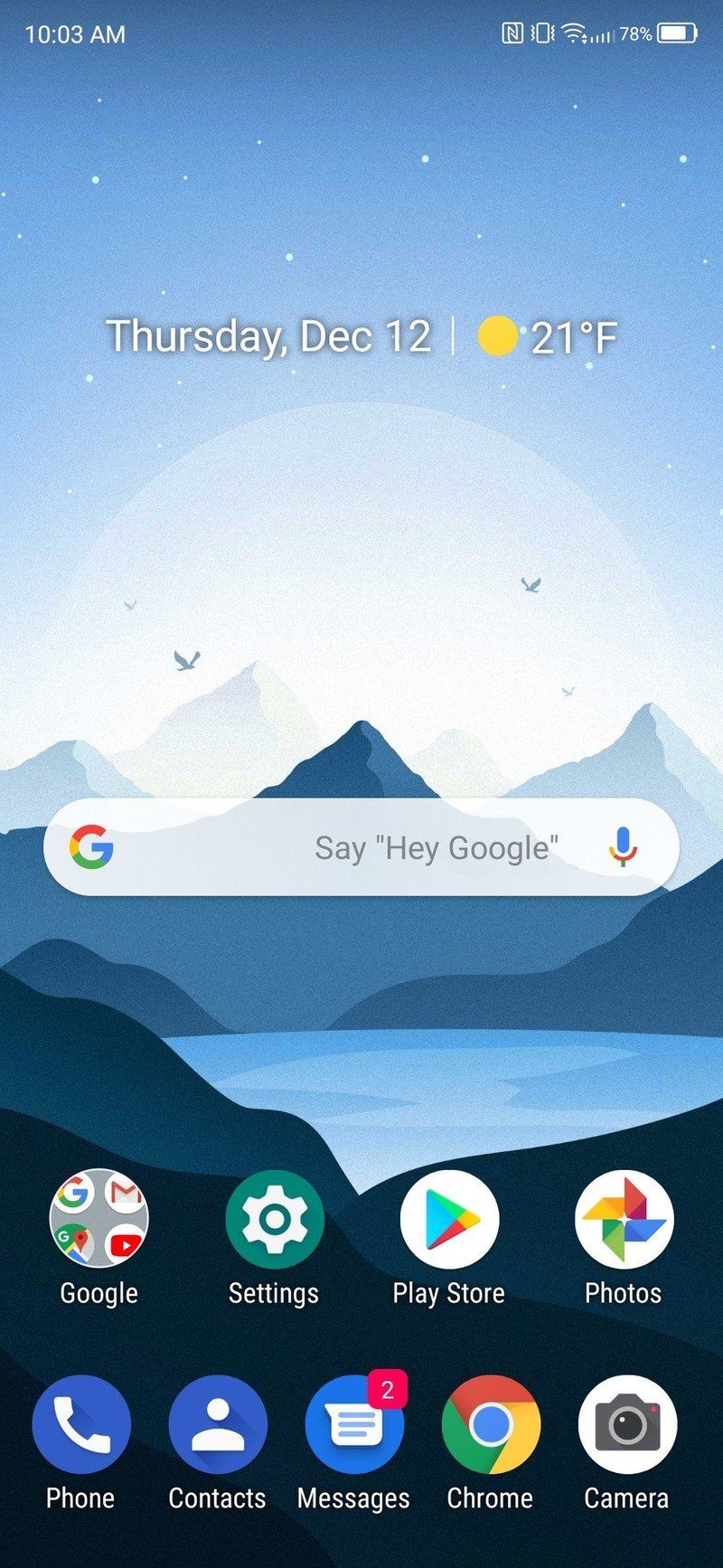The smartphone screenshot shows the device's screen at 10:03 a.m., with a battery level at 78%, and a cellular signal strength of 4 out of 5 bars. The home screen features a serene wallpaper depicting a blue sky that gradually lightens as it approaches the horizon, framed by distant mountains and a small lake in the foreground. Birds soar through the sky, adding a touch of life to the tranquil scene.

A white search box positioned prominently at the top of the screen features the Google logo, accompanied by the prompt "Say Hey Google" and a microphone icon to the right.

Below the search box, two rows of app icons are neatly arranged. In the top row, from left to right, are icons labeled "Google," "Settings" (illustrated with a gear), "Play Store," and "Photos." In the bottom row, the icons are labeled "Phone," "Contacts," "Messages," "Chrome," and "Camera."